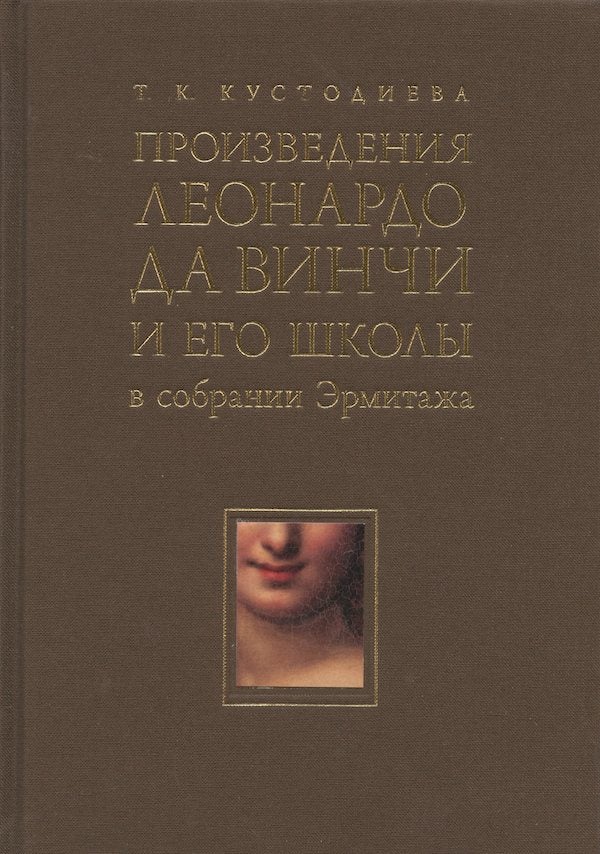The image depicts the front cover of a large, textured, brown hardcover book adorned with gold lettering in a language that is not English, possibly Russian, featuring some characters that resemble those in the English alphabet. At the top, there is a person's name consisting of the initials T.K followed by what appears to be the surname K.Y.C.T.O.A.N.E.B.A. Below this, an unreadable title in similar gold lettering spans multiple lines. Towards the center bottom of the cover, within a gold-outlined square, there is a small photograph that showcases part of a woman's face—from the bridge of her nose down to her neck—cropped in such a way that her eyes and part of her right cheek are not visible. The woman has red lips turned slightly upwards in a closed-mouth smile.